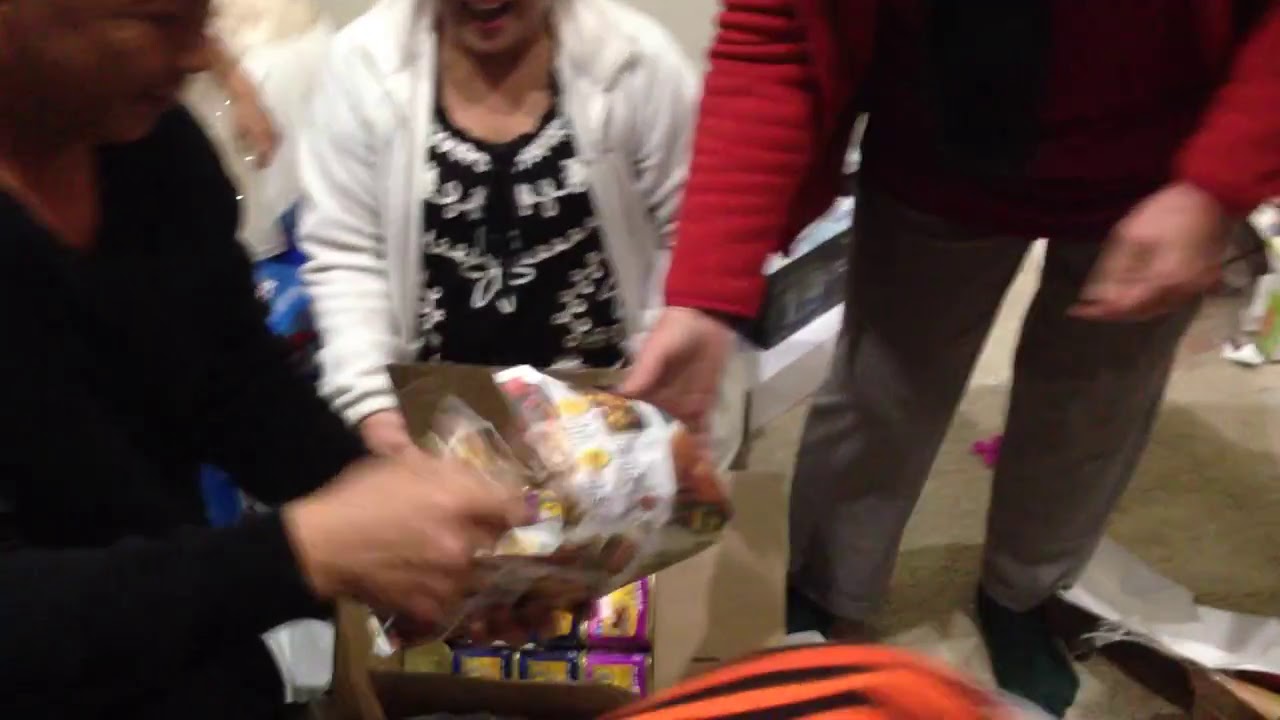In the photograph, several people are gathered in a semi-circle, all involved in opening an object, possibly a packaged food item. At the center stands an older woman, identifiable by her smiling lower face. She wears a white cardigan over a black and white shirt. To her left, a person in a dark long-sleeved sweater is seen handling the object, while to her right, another individual wearing a red long-sleeved jacket with gray pants and black socks also holds onto the item. The immediate surroundings show a bit of clutter, including an orange item, a white cardboard box, various plastic bags, paper, and small purple and blue objects scattered on the tan-colored floor. Behind the main group, a person in a white jacket and black dress can be seen holding a box filled with cans, adding to the scene's bustling atmosphere. A brown pillow is also visible in the background.